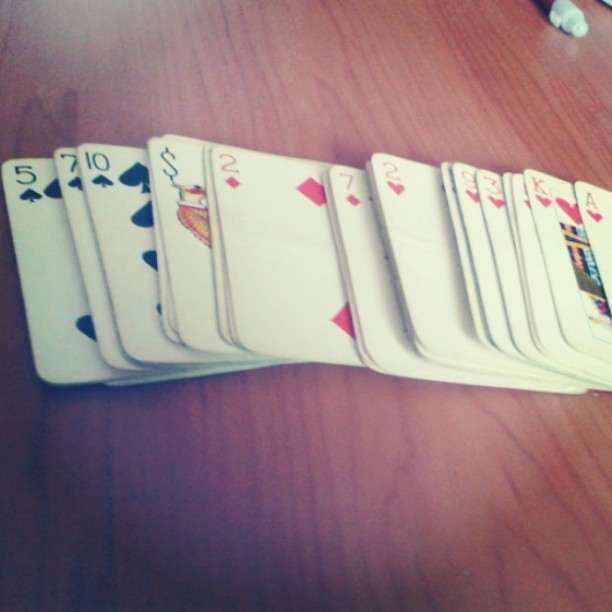A wooden table serves as the backdrop for a meticulously arranged deck of cards, spread out in a slightly fanned manner but still maintaining a somewhat stacked formation. The sequence begins with the Ace of Hearts, followed by the King of Hearts, and continues in suit order: Hearts, Diamonds, Spades, and Clubs. Central to the array, bridging the gap between the red and black suits, is the Joker card included with the deck. Although not all individual cards are fully visible due to their overlapping layout, the organized pattern is discernible. The scene suggests imminent action, possibly a person, hinted as female, preparing to shuffle the cards. 

In the upper right-hand corner of the photograph, a blurry object is visible, though its details remain indistinguishable. The lower left-hand corner of the image is notably darker than the rest of the scene, creating a subtle gradient. The lighting indicates either daytime or a strong overhead light source illuminating the setup.